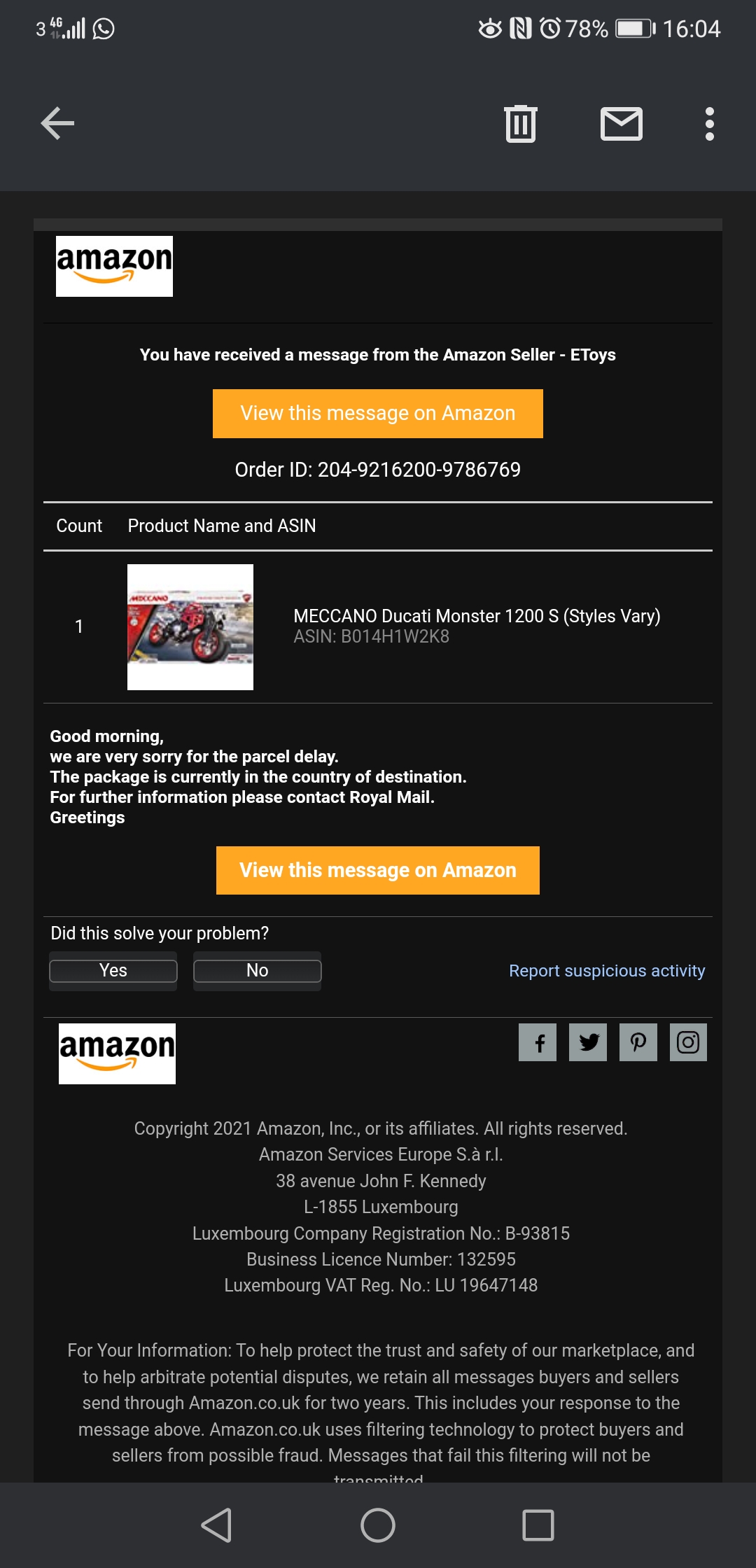The image displays an email from Amazon, viewed in a mobile email application set to dark mode. The email is a communication from the Amazon seller "eToys," informing the customer that they have received a message. The top of the email features a button labeled "View the message on Amazon."

It provides specific details about the order, including the order ID, the product name (Ducati Monster - a motorcycle), the quantity (one), and the ASIN. The body of the email contains a message from the seller expressing apologies for a parcel delay. The message states, "Good morning, we are very sorry for the parcel delay. The package is currently in the country of destination. For further information, please contact Royal Mail. Greetings."

At the end of the message, there’s another button to view the message on Amazon, followed by a query, "Did this solve your problem?" with "Yes" and "No" options.

The email concludes with general Amazon information including social media links, copyright details, business registration address, and a note. The note informs users about Amazon's communication policies, stating: "To help protect the trust and safety of our marketplace, and to help arbitrate potential disputes, we retain all messages buyers and sellers send through Amazon.co.uk for two years. This includes your response to the message above. Amazon.co.uk uses filtering technology to protect buyers and sellers from possible fraud. Messages that fail this filtering will not be transmitted."

Overall, the detailed email provides comprehensive information about the delayed package and underscores Amazon's commitment to secure and trustworthy transactions.